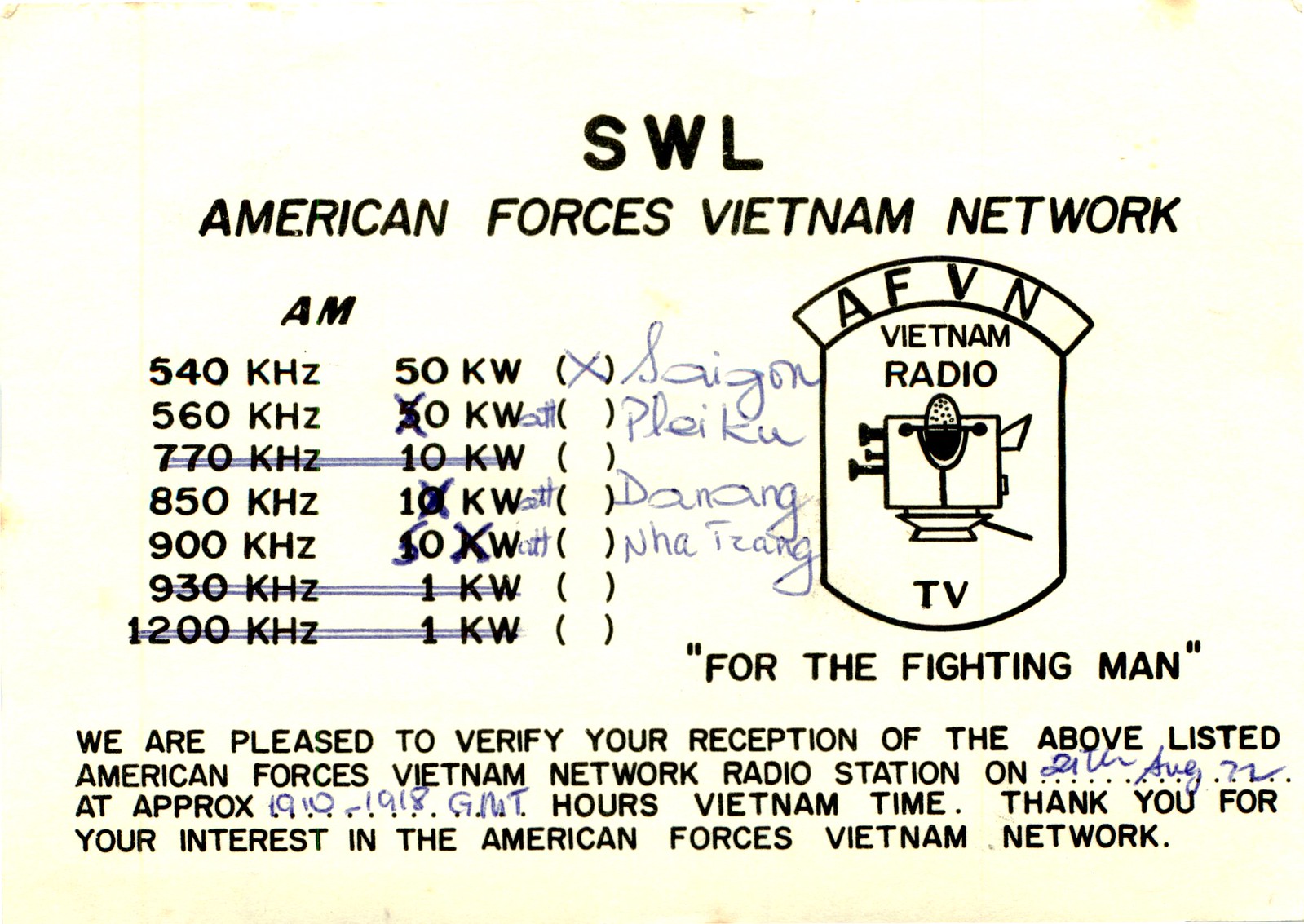This image showcases an aged yellow card, titled "SWL" at the top, with black lettering and sections of blue ballpoint pen markings. It features detailed information about the American Forces Vietnam Network (AFVN) radio stations. Below the main heading, "American Forces Vietnam Network" is prominently displayed, followed by a list of AM radio frequencies: 540 KHz, 560 KHz, 770 KHz, 850 KHz, 900 KHz, 930 KHz, 1200 KHz, with power outputs noted as 50 KW, 10 KW, and 1 KW. 

A faded illustration of a film camera and a television microphone is placed on the middle left, marked with "AFVN Vietnam Radio" and the phrase "For the Fighting Man." The card includes spaces where frequencies have been crossed out and annotated with locations such as Saigon, Pleiku, and Da Nang. The card serves as a confirmation of reception for listeners, expressing appreciation for their interest in the AFVN radio stations. The colors are noted to be predominantly faded yellow, with accents of white, blue, and black.